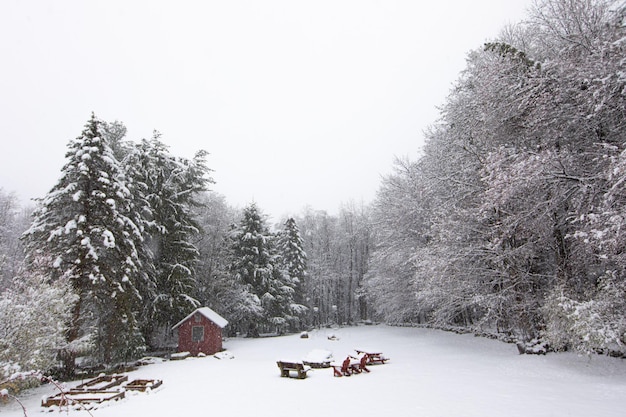The photograph captures a picturesque winter scene set in a snow-covered forest. Dominating the landscape are towering trees blanketed in snow, forming a semicircular pattern from one side of the frame to the other. To the left, a mix of bare-branch trees and snow-laden evergreens creates a stark contrast, while to the right, lush pine trees peek out from beneath their snowy covering. The ground is completely white, hiding any trace of earth beneath a thick layer of snow. 

In the center of the image, there is a clearing with an arrangement of benches and chairs encircling what appears to be a fire pit, all dusted with snow. This setup evokes a sense of a communal gathering spot, now frozen in winter’s grip. To the left side of the clearing, there is a small garden area, demarcated by wooden borders, also buried under snow.

On the bottom right corner of the picture, sits a tiny red cabin or shed with a snow-covered roof. This structure, possibly used for storage or as a small retreat, adds a charming touch to the wintry landscape. In the background, just barely visible, are hints of vehicles or perhaps a snowmobile, suggesting outdoor activity in this serene and remote setting.